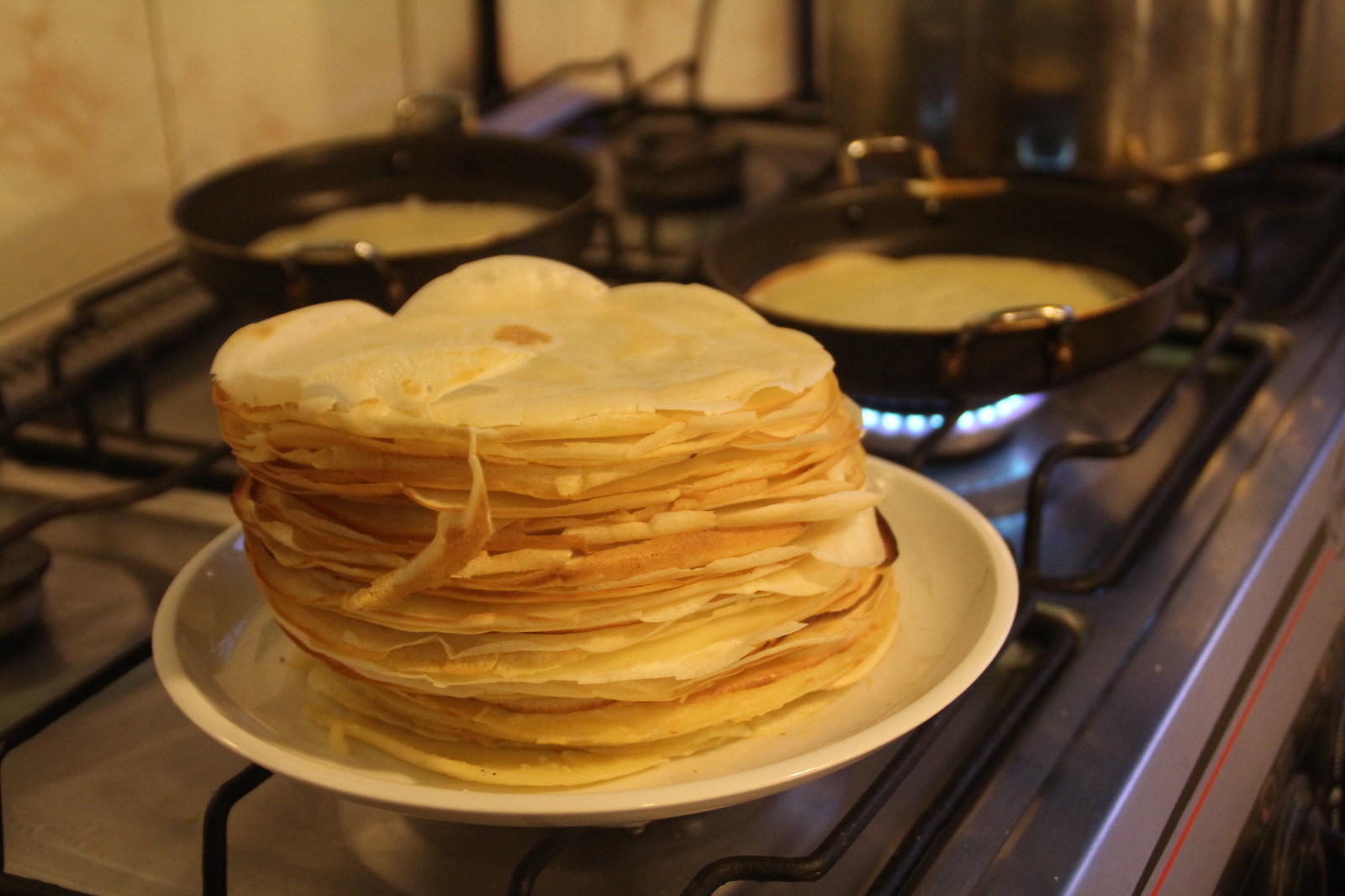The photograph shows a gas stove with black grates over the large burners, which support two black skillets with silver handles. Each skillet contains a beige batter with hints of brown. In front of the background skillets is a white plate on the front burner, holding a meticulously stacked pile of thin crepes. The crepes have a golden exterior with some browning in the center and darker spots, indicating a perfectly cooked texture. The lighting in the kitchen gives the scene a slightly yellowed tone, emphasizing the warm, inviting atmosphere as freshly made crepes are prepared.